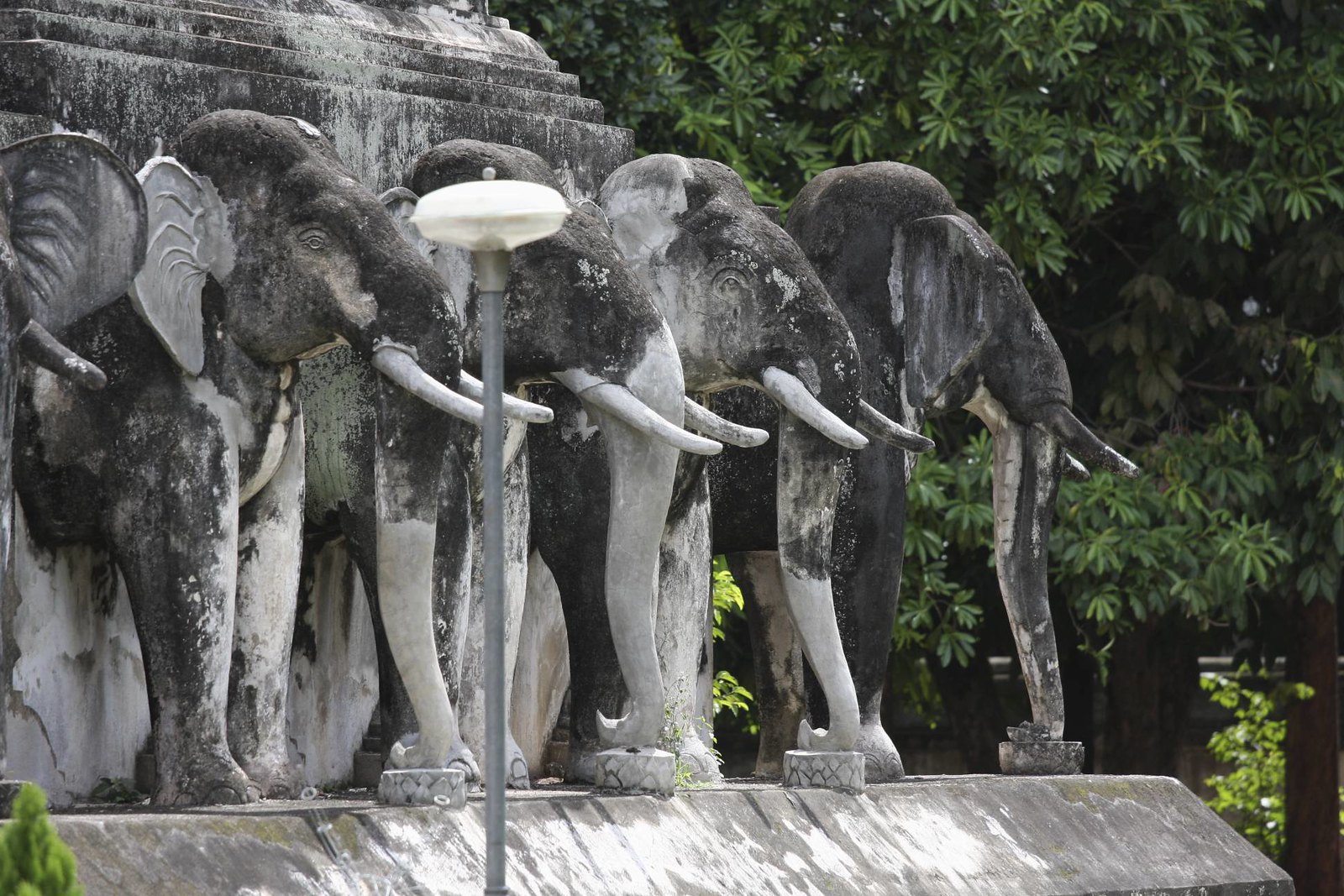The photo captures an angled partial view of a monument adorned with life-sized stone statues of elephants at its base. The elephants, originally white like the monument itself, have turned varying shades of dark gray and black due to weathering and age. Each elephant has white tusks, large ears, and trunks that are curved downwards under the base of the monument. Some statues show signs of wear, with pieces of their ears missing, but overall, they remain well-maintained and exhibit a natural stone texture, highlighted by patches of moss and organic growth. Behind the monument stands a structure featuring an arched section and indentation near the top, also made of stone. In the background, a grove of green trees can be seen, and in the left-center area of the photo, a thin silver lamppost with a light on top is visible. The bottom left corner of the image features leaves from an overhanging tree, adding to the scene’s natural ambiance.